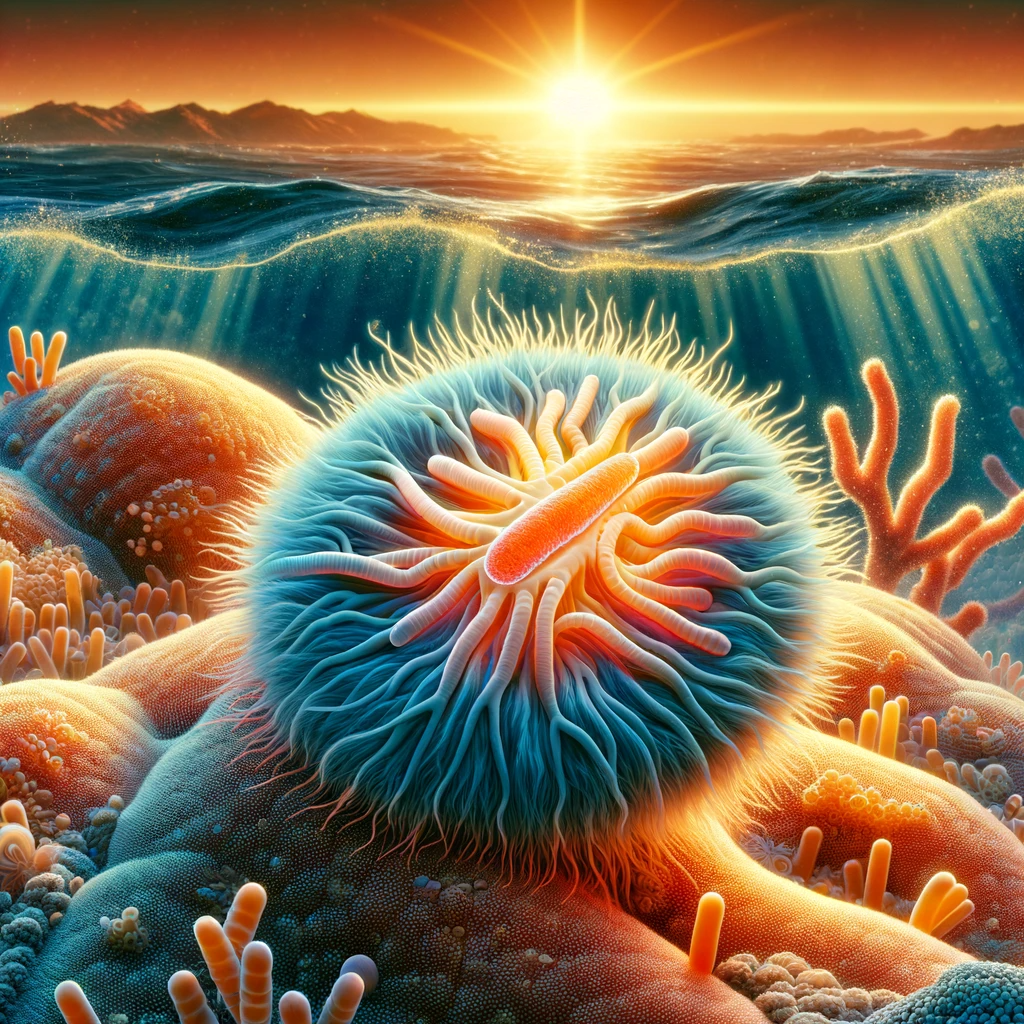In this fantasy-style, highly detailed digital illustration, we observe a mesmerizing underwater scene reminiscent of microscopic life. The image opens with a contrasting dark outline that represents the sky, gradually shifting to an orange glow indicative of a setting sun. Central to the top section is a radiant white and orange orb, complete with fiery flares, symbolizing the sun. On the left, the sun casts orange highlights on a rugged line of mountains, while a smaller silhouetted mountain range appears on the right. Beneath this landscape, the surface of the ocean is depicted with dramatically agitated, teal-blue water, marked by dark edges and brilliant highlights where the sunlight pierces through.

Diving below the water’s surface, golden rays penetrate the ocean, creating a cross-sectional view teeming with fantastical underwater life. The seabed is strewn with orange mounds featuring blue highlights, suggesting a vibrant coral reef environment. Dotting these mounds are bright orange pill-shaped creatures and similarly colored kelp-like organisms, each adding to the scene's surreal detail. At the center of this intricate tableau is a peculiar mass of blue tendrils, resembling a tangled congregation of worms. Nestled within this mass is a prominent pill-shaped object, strikingly bright orange with a light-blue halo, vaguely carrot-like in its appearance. This captivating composition seamlessly merges realistic oceanic elements with the enchanting and magnified view one might expect under a microscope, thus blurring the lines between reality and a fantastical underwater world.